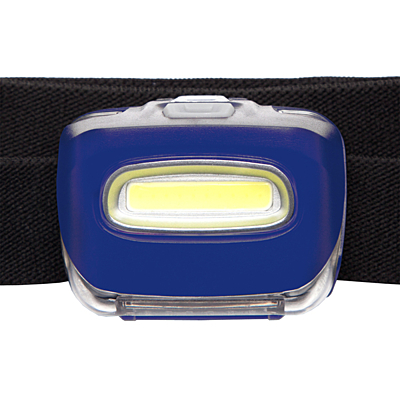The image depicts a detailed, close-up color photograph of a blue plastic case, viewed in landscape orientation. The case is horizontally rectangular with sharply rounded corners that flare towards the top. The top and bottom quarters of the image feature white spaces, while the middle section prominently displays the blue object. The case appears to be constructed from a shiny silver metal that frames a blue plastic surface.

In the center of this blue surface, there is an elliptical, horizontally-oriented oval shape, outlined with the same silver metal. The interior of this oval shape glows yellow, possibly due to an internal light source, and seems intended for writing or labeling. The case also features two clear handles, one at the top and another at the bottom, suggesting the case can be opened from either end. A cylindrical hinge at the bottom likely helps to secure the lid when opened.

The background behind the case consists of a black, textured material resembling the texture of gym shorts, with a strap or cloth-like appearance visible. Additionally, the photograph shows part of a plug-in portion along the bottom edge of the case. The overall presentation is in a photographic realism style, emphasizing the detailed textures and colors of the objects depicted.